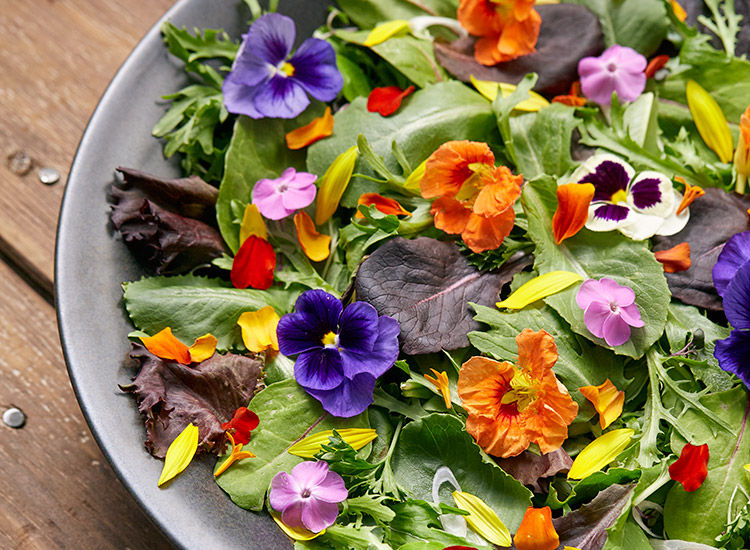A top-down view reveals a light gray bowl resting on a dark brown wooden table, partially visible on the left. Inside the bowl, a mix of green leaves and dark purple leaves form a classic salad mix. Scattered throughout the greens are an assortment of colorful, edible flowers. Among them are several dark purple flowers, some with five petals and a white center, others with a yellow center. There are also vibrant orange flowers, each with four or five large, curvy petals and a prominent yellow center. Additionally, some light pink and white flowers add to the visual feast. The salad also features some yellow leaves, enhancing the dish's variety and coloration.